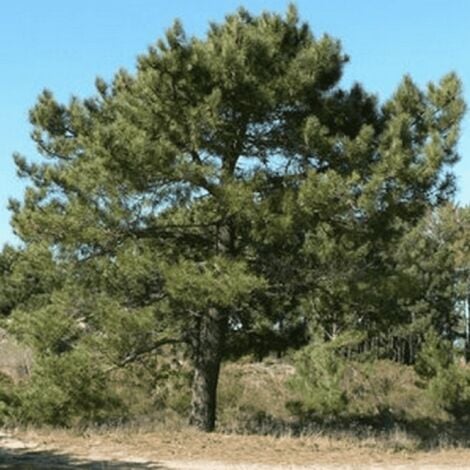The photograph depicts a scene from nature, featuring a prominent and bushy pine tree standing by the side of a public road, positioned at the center of the image. This short, yet wide tree is characterized by its round outline and long green needles, with a thick trunk that contrasts with its more slender branches. The ground below the tree is scattered with dead brown pine needles, contributing to the dry and somewhat neglected appearance of the environment.

The landscape around the tree includes several other smaller bushes and additional trees dispersed in the background, indicative of a natural, untamed setting. The terrain is mostly flat, except for a small hillside where the pine tree stands. The ground, predominantly brown and tan, shows little sign of grass, suggesting it hasn't seen rain in a while.

Above, the sky is a clear, vivid blue with few or no clouds, enhancing the outdoor atmosphere of the scene. The photograph is a square format, capturing the essence of a dry, brush-filled area that has not been carefully gardened or manicured. The colors span a range of greens, browns, tans, and blues, creating a serene yet somewhat arid landscape devoid of urban elements.